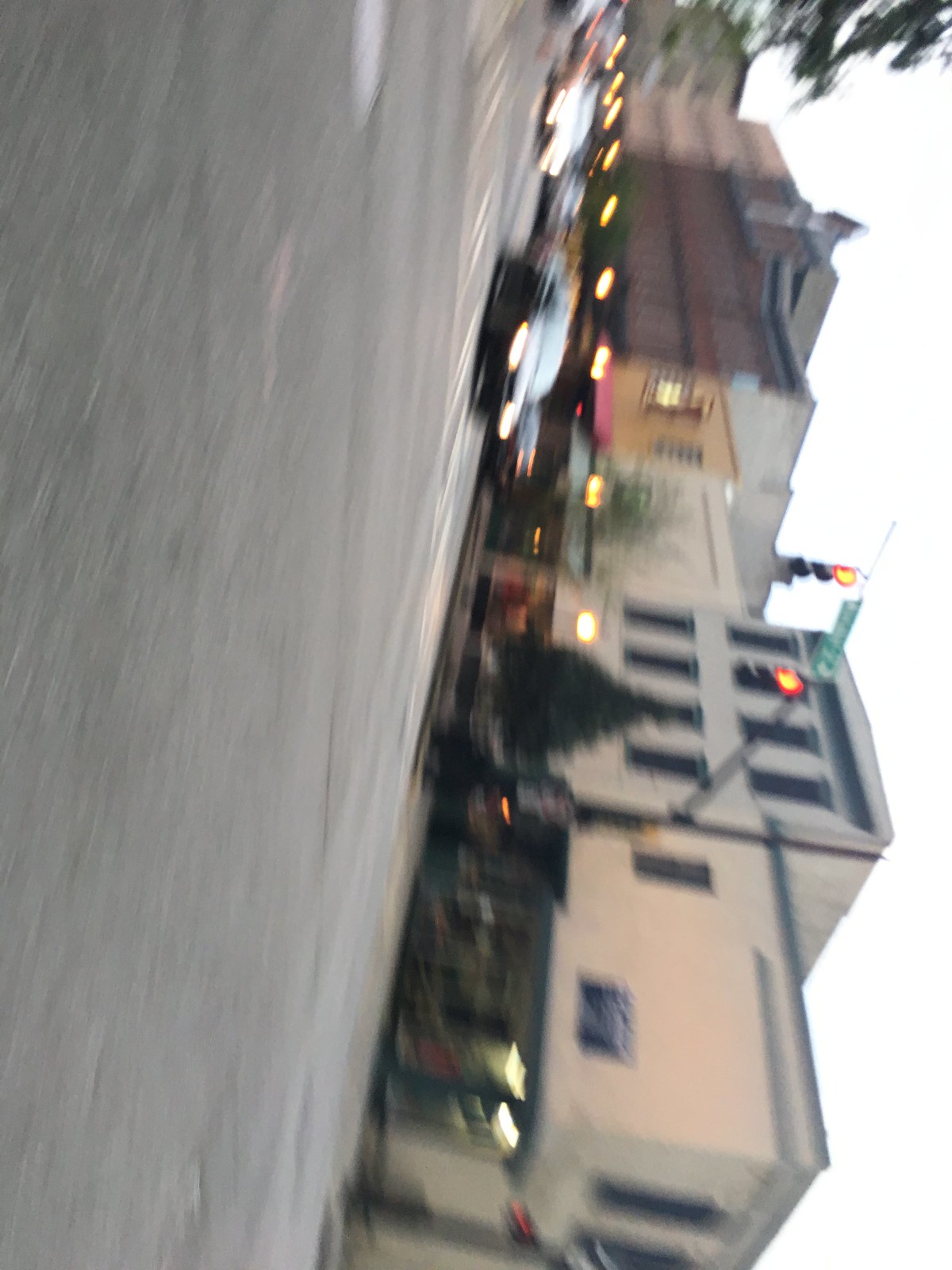This photograph depicts a disorienting, blurry daytime scene of a town street. Captured at a sideways angle, the tops of the buildings are aligned to the right. Two cars appear to be speeding towards the viewer, their images distorted by the blur. The left portion of the photo is dominated by angled pavement, while the right side showcases a row of multi-story buildings interspersed with trees, including a recognizable pine tree. Various buildings rise to three and four stories, adding to the urban setting, and there are indistinct streetlights dotting the scene, contributing to the overall motion and blur of the image.